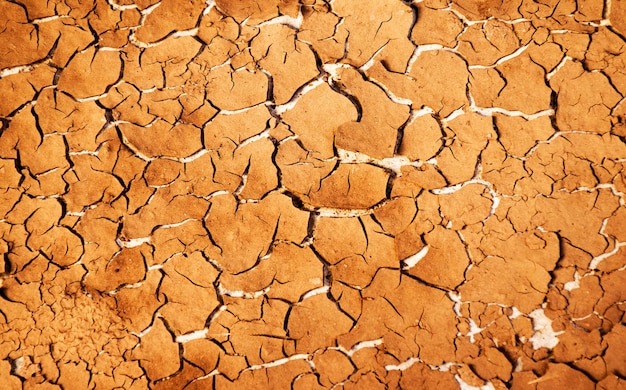This detailed close-up image captures the arid, cracked ground of what appears to be a dry lake bed, likely situated in the Mojave Desert. The photograph, taken from a top-down perspective, showcases a vast expanse of desiccated earth. The terrain consists of parched, ochre-colored clay that has fractured into numerous irregularly shaped sections. These sections vary in size, with larger unbroken pieces predominating in the center and more fragmented, sand-like pieces towards the edges.

Scattered across the surface are terracotta-hued rocks, some chipped into smaller pieces due to natural wear and tear. Patches of a pale, white underlying surface are visible through the cracks and where some rocks are missing, particularly notable in the lower right corner of the image. This detailed texture shot, devoid of any trees, humans, or animals, offers a raw, minimalist glimpse into the stark beauty of a dry, cracked desert floor, making it a potential candidate for graphic design applications.